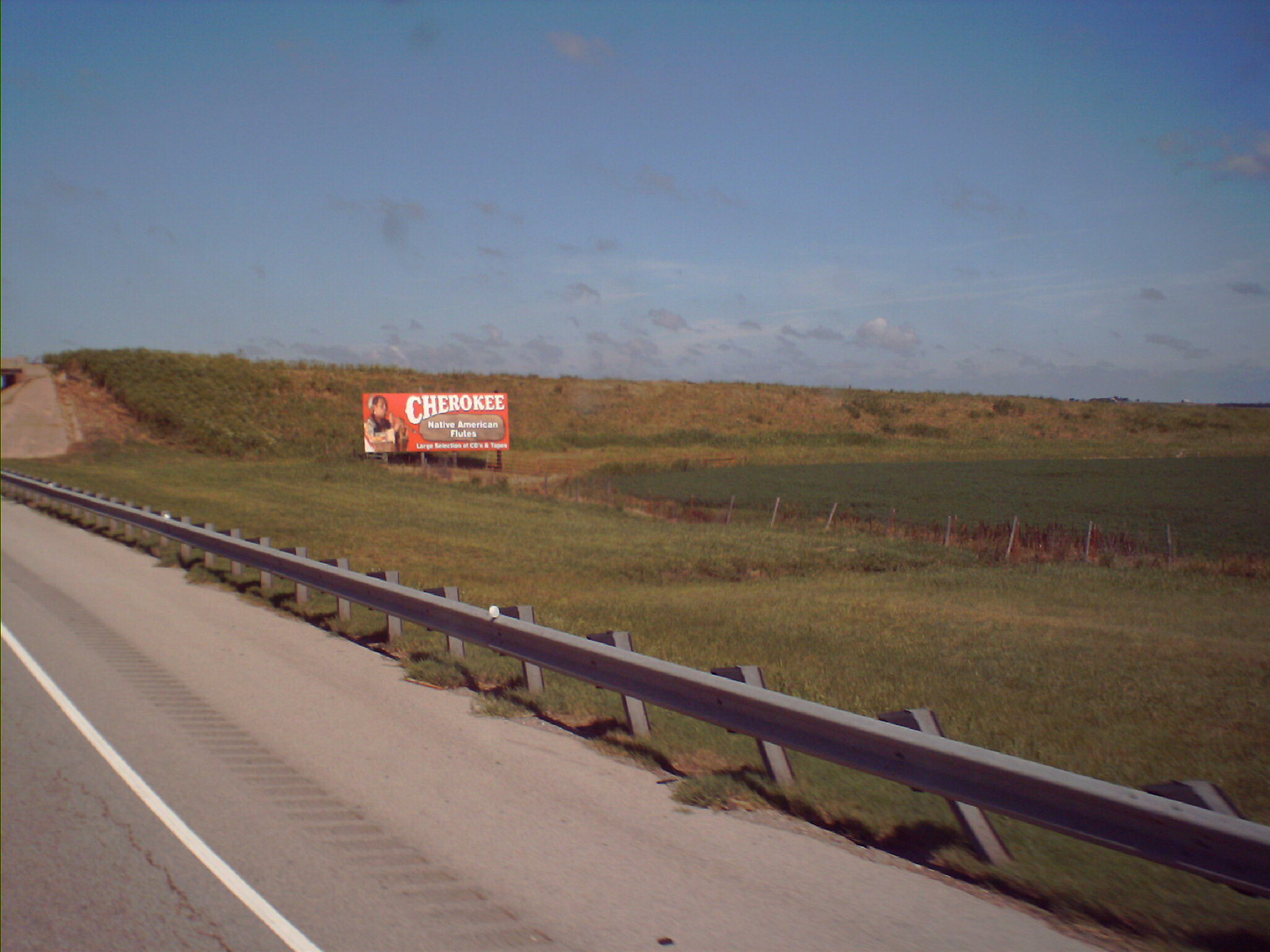The image, taken from a car on an underpass road, captures a scenic outdoor view featuring a grayish-blue sky dotted with small gray clouds. The horizon is dominated by a hill blanketed with rows of green and yellow bushes. In the foreground, a sprawling green grassy field stretches alongside the roadside, partially enclosed by a chain-linked fence. A prominent, vibrant orange billboard with bold white text reading "Cherokee" and an illustration of a Native American man stands at the edge of the field, next to a darker green section that resembles a farm field. This fenced-off area is seen before a metal guardrail and a white-striped roadway, which is further bordered by safety bumps designed to alert drivers. Above the roadside, a bridge and steel concrete ramp frame the top of the image, suggesting that the photograph was taken from a lower level roadway looking towards an overpass.